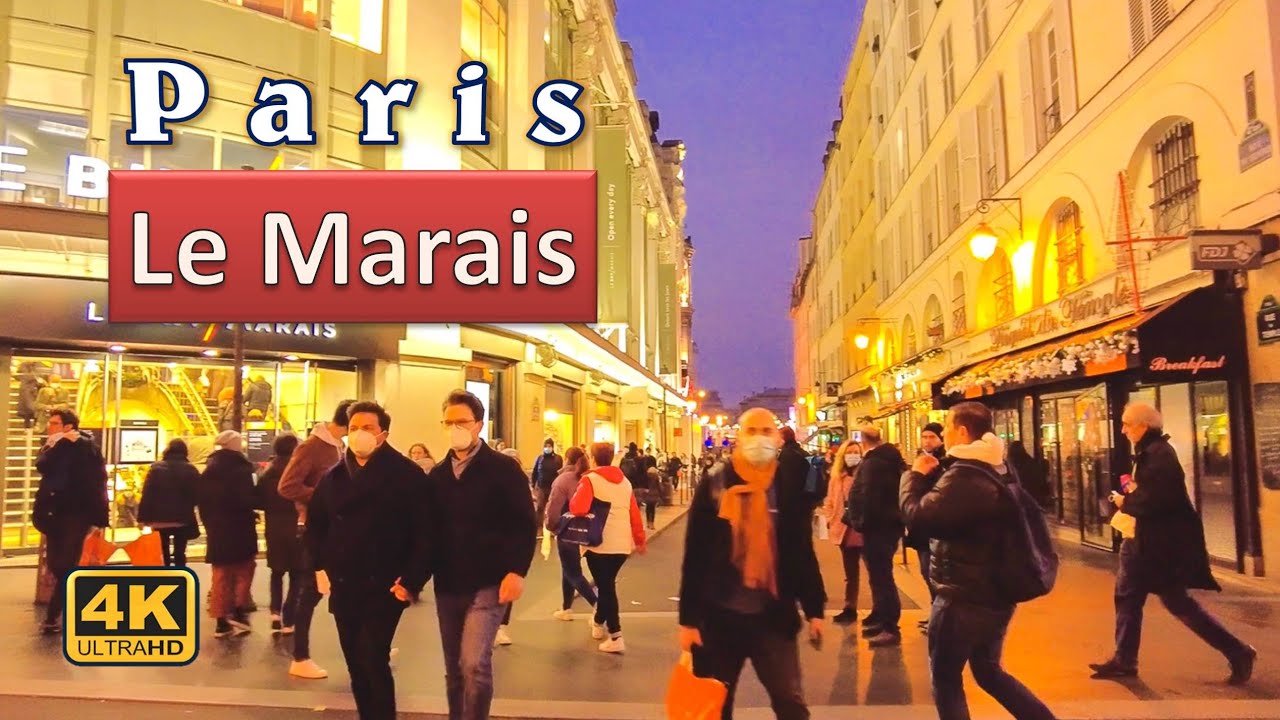This color photo captures a vibrant, busy street scene at night in the Le Marais district of Paris. The foreground is filled with people of all ages and genders, most wearing dark jackets and face masks, walking through the brightly lit street. Enhancing the scene are buildings on either side, bathed in a golden yellowish hue, with a hint of orange on the ground. The upper part of the image reveals a sliver of the sky in a mesmerizing purplish-blue tone, suggesting dusk or evening. In the top left corner, white letters spell out "Paris," with "Le Marais" displayed below in a red banner, accompanied by "4K Ultra HD." Among the pedestrians, a bald man slightly out of focus stands out, adorned with a red scarf and carrying a matching shopping bag. Two men to the left hold hands; one dressed all in black, the other with glasses and dark hair. The streets are alive with the glow of amber streetlights illuminating the high-end shops on this smooth, reflective boulevard, creating a warm and inviting atmosphere.